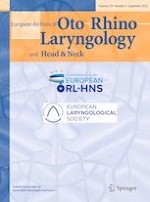The image depicts the cover of a small, vertically rectangular book, likely a college textbook centered around the subject of otorhinolaryngology, which is the study of diseases of the ear, nose, and throat. The cover features a blue binding on the left side and another blue binding extending halfway across the top. At the top, there's an orange rectangle with large blue letters spelling out "Otorhinolaryngology." Below the orange rectangle, two white rectangles are positioned side by side against a light blue background. Further text on the cover includes references to "European ORL" and "HNS," as well as a mention of a European society, signifying its specialized and academic nature. The bottom half of the cover showcases a light blue and white pattern, possibly swirls or abstract designs, contributing to the overall subtle aesthetic of the book.